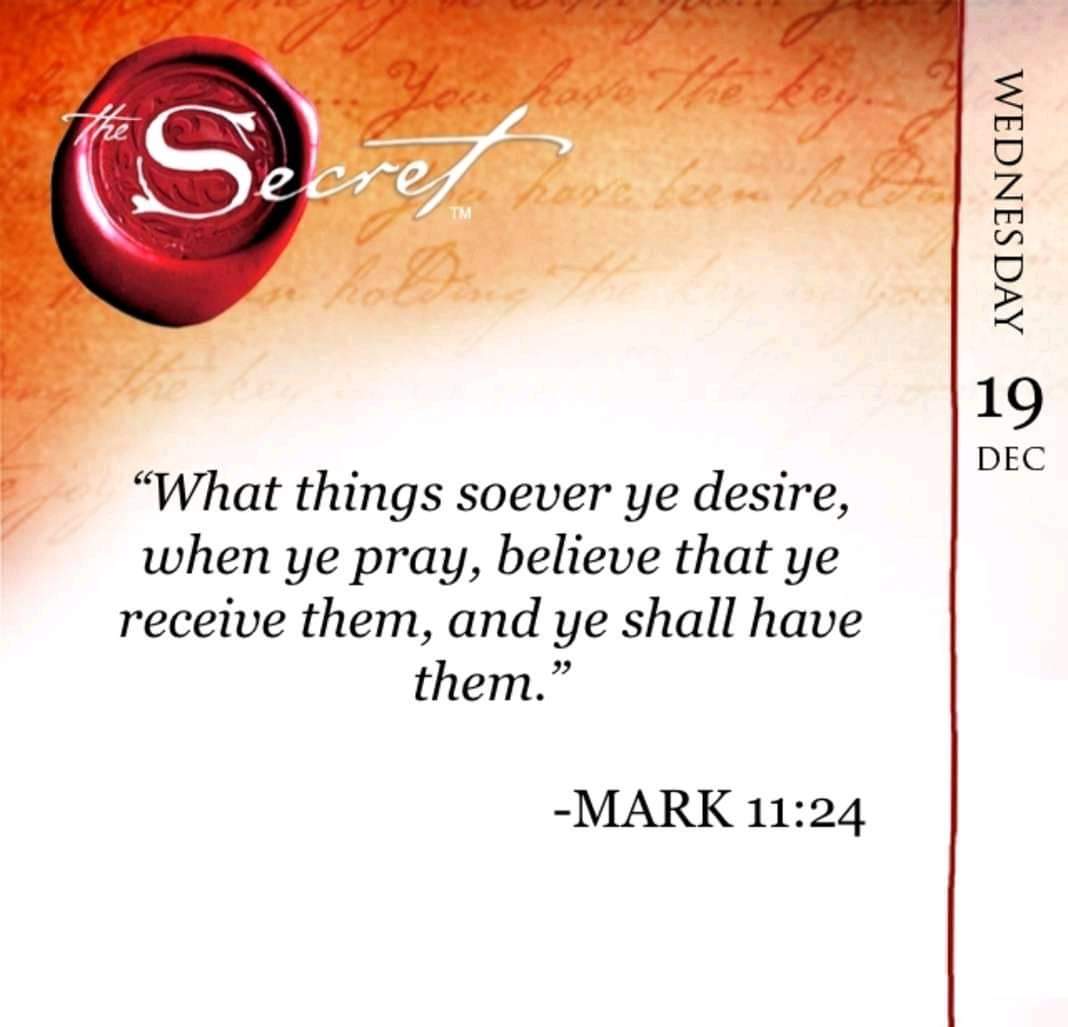The image is a detailed book cover for "The Secret." It features a Bible verse, Mark 11:24, which reads, "What things soever ye desire, when ye pray, believe that ye receive them, and ye shall have them," in black text against a background that transitions from a burnt orange at the top to white at the bottom. In the top left corner of the cover, there is a red circular wax seal containing the title "The Secret" with a prominent "S" in the center, further signified by a TM (trademark). The background features cursive text that gradually fades out as it reaches the bottom of the image. Along the right side of the cover, the word "Wednesday" is written sideways, followed by "19 DEC" indicating the date, December 19th.